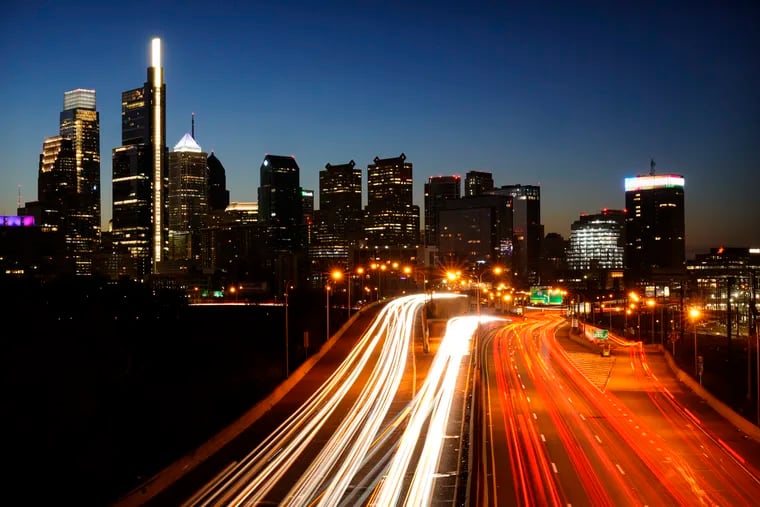The photograph captures a vibrant cityscape viewed from an elevated perspective, either by drone, helicopter, or high vantage point. It’s taken at twilight—either just before sunrise or just past sunset, creating a blend of natural and artificial light. A prominent highway runs across the bottom of the image, divided into multiple lanes. The long exposure reveals streaks of light from moving vehicles: bright white lines from headlights on the right and red taillight trails on the left. Midway along the highway, a few signs are visible but unreadable. The city beyond the highway boasts an array of skyscrapers, with their illuminated windows piercing the night. Towards the center-left, the sky transitions from a deeper blue to a lighter hue, influenced by the twilight. Off to the far left, the buildings are adorned with distinctive pink and three purple lights, adding a splash of color to the urban scene. The overall palette includes orange, red, yellow, white, black, and green, reflecting the dynamic interplay of night and city lights. The scene captures the urgent, bustling life of the city in a single, striking snapshot.